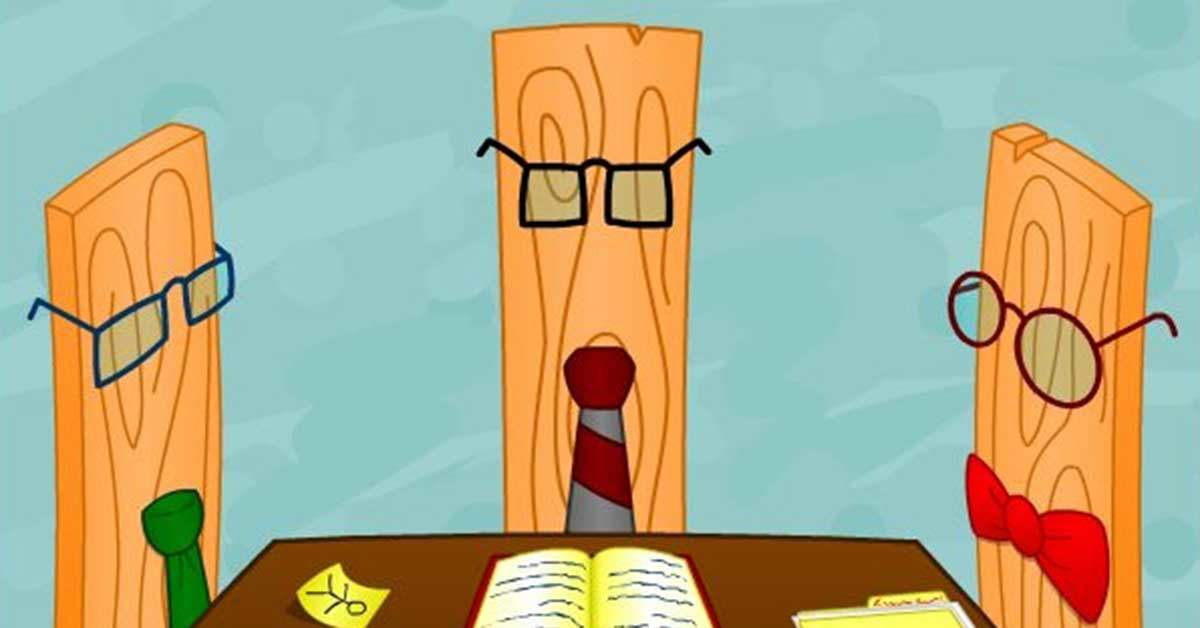In this cartoon-style drawing set against a light blue background, three anthropomorphic vertical wooden planks are seated around a dark brown rectangular table. Each plank is adorned with a unique pair of eyeglasses and a distinct type of neckwear. The plank on the left wears blue rectangular glasses and a green tie, the center plank dons black square glasses with a burgundy and gray striped tie, and the plank on the right sports brown glasses with a bright red bow tie. The table itself is organized with three items: a yellow post-it note with a stick figure drawing on the left, an open red book with scribbles in the center, and a file folder alongside another post-it note on the right. The wooden planks are distinctly tan-colored, giving them a natural wood appearance, and they seem to be studying the materials on the table, creating an impression of a serious meeting scene crafted in a whimsical, cartoonish manner.